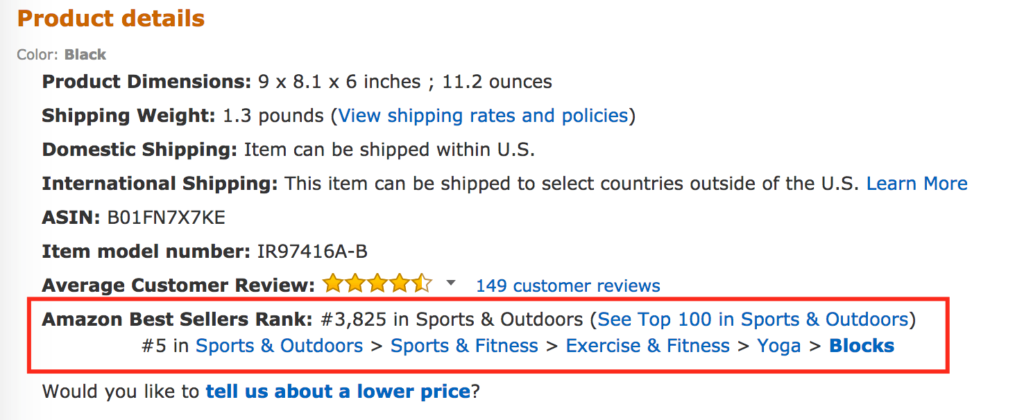This image shows a detailed product listing on Amazon. In the upper left corner, "Product Details" is displayed in an orangey-brown color. The listing specifies the product color as black and includes the dimensions: 9 by 8.1 by 6 inches, with a weight of 11.2 ounces. The shipping weight is noted as 1.3 pounds. 

Below the dimensions, there is a link labeled "Shipping rates and policies" in blue text. The product is available for domestic shipping within the U.S., and international shipping to select countries outside the U.S. More details can be found via the "Learn more" link in blue.

The ASIN for the product is B01FNSOF7X, and the model number is IR97416A-B. The average customer rating is 4.5 stars based on 149 customer reviews. Highlighted in red is the Amazon Best Sellers Rank: #3,825 in the Sports & Outdoors category, and #5 in the Sports & Fitness > Exercise & Fitness > Yoga Blocks subcategory. 

There is a prompt for users to inform Amazon about a lower price for the product, with the link "tell us about a lower price" also in blue. The highlighted links and the entire Amazon Bestseller rank section are enclosed within a red rectangle, suggesting this image may be used for educational purposes.